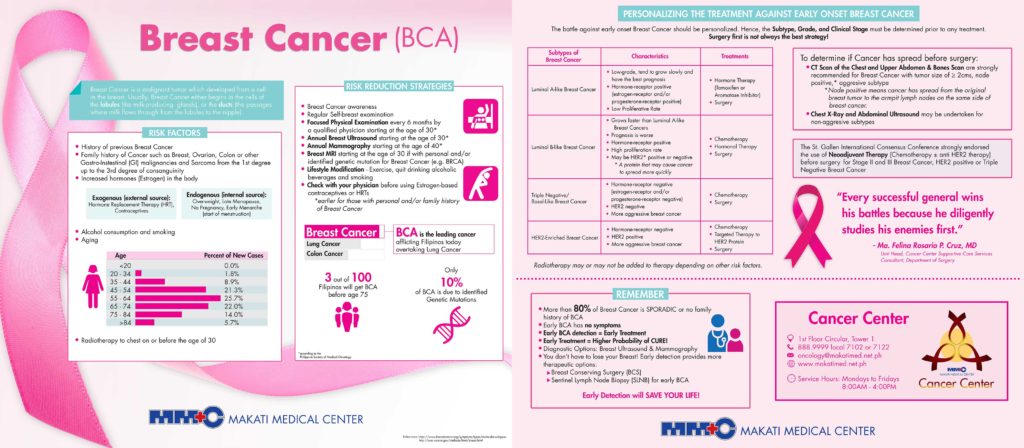Here's a detailed and cleaned-up caption for the image:

---

"This infographic from Makati Medical Center focuses on breast cancer awareness. The entire visual is adorned in shades of pink, a color symbolizing breast cancer awareness. The background and the charts are uniformly pink. The content includes comprehensive details on the symptoms of breast cancer, common risk factors, and the influence of elevated estrogen levels in the body. Additionally, it highlights the significance of a family history of cancers, including breast, ovarian, colon, and other gastrointestinal malignancies, extending from first-degree to third-degree relatives. 

The infographic features a specific chart depicting the age distribution of new breast cancer cases. The age range starts from 20 years and extends beyond 84 years, indicating the percentage of new cases within each age group. Notably, the percentage for ages 20 to 34 is marked at 1.5%. However, this particular chart is slightly blurry, making it difficult to see the finer details."

---

This caption provides a comprehensive and clear overview of the image content while ensuring all key points are mentioned.